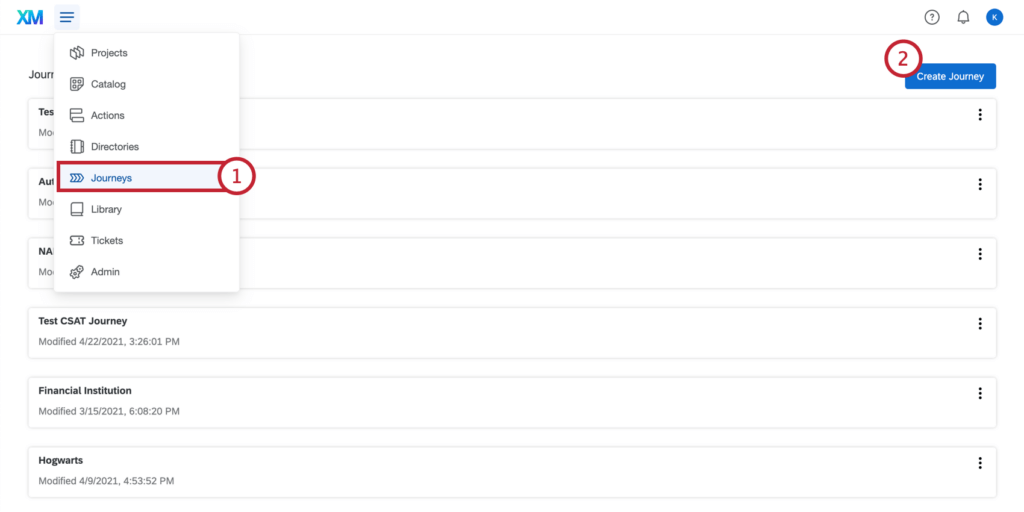The image showcases a digital interface displaying a structured dashboard. The left side of the image features a navigation panel with menu items such as Projects, Catalog, Actions, Directions, Journeys, Library, Tickets, Admin. Below the menu, there are several entries listed, including "Test CISAR Journey," which was modified on March 4th and April 22nd, 2021. The timestamp for the latest modification is recorded as 3:26:01 PM. Another entry, titled "Financial Institution," was last modified on March 15th, 2021, with a timestamp of 6:08 PM. Additionally, an entry labeled "Hogwarts" shows its last modification date as April 9th, 2021, with a timestamp of 4:53 PM. This organized layout allows for efficient management and review of various projects and actions.